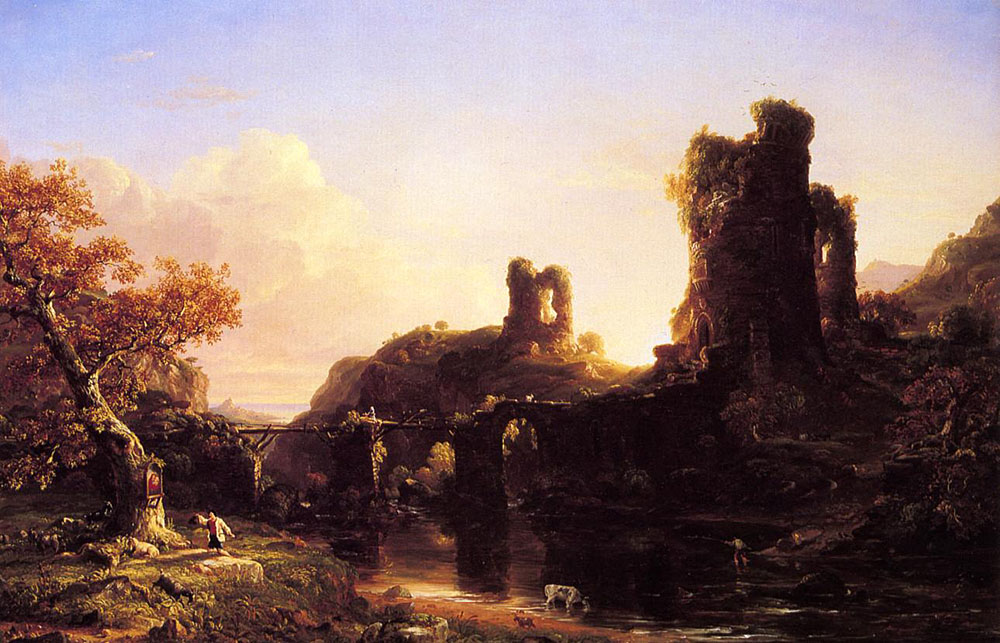This painting, titled "The Decline of Civilization," is an intricate and highly detailed landscape that reflects a surreal yet realistic art style. Dominating the foreground is a wide river or large creek, its water shimmering with light. A cow stands at the water's edge, drinking, while to the left, a patch of green grass and rocky soil supports a tree adorned with vivid yellow and orange leaves. The tree, adjacent to a small shrine, has a man in a white coat standing in front of it, possibly holding a lantern. The tree's bark and the surrounding dirt path are rendered with striking realism.

Behind the tree runs an old, partially degraded stone bridge, its remaining arches and temporary wooden boards hinting at former glory. Beyond the bridge, decrepit turrets and towers, remnants of a castle covered in vines and ivy, rise from the rocky, brown landscape. In the sky, soft clouds are scattered across a blue expanse, with hues of pink and yellow suggesting a sunny, light-filled day. The sunlight reflects off the landscape in a way that enhances the painting's depth and detail.